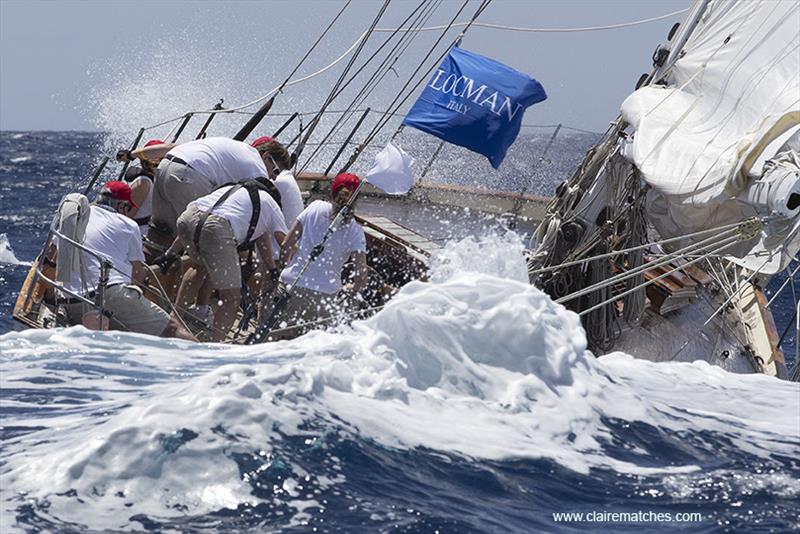This professional, full-color square photograph captures an intense moment during a daytime sailing race on a rough ocean. Dominating the scene is a yacht battling towering waves, with white foam crashing over its sides. The vessel appears to be sharply turning to the right, compelled by the force of a significant wave on its starboard side. To counterbalance this, six crew members are strategically positioned on the yacht's port side, seemingly applying their combined weight to keep the yacht steady. Each crew member is attired in uniform outfits consisting of khaki shorts, white t-shirts, and red baseball caps. The intensity of the moment is augmented by the visible wind, which is fully unfurling a blue flag located at the yacht's stern. This flag prominently displays the word "LOCMAN" in white, uppercase letters, with "ITALY" noted below. Additionally, in the lower right-hand corner of the image, the website "www.clarimatches.com" is clearly visible in white lettering.